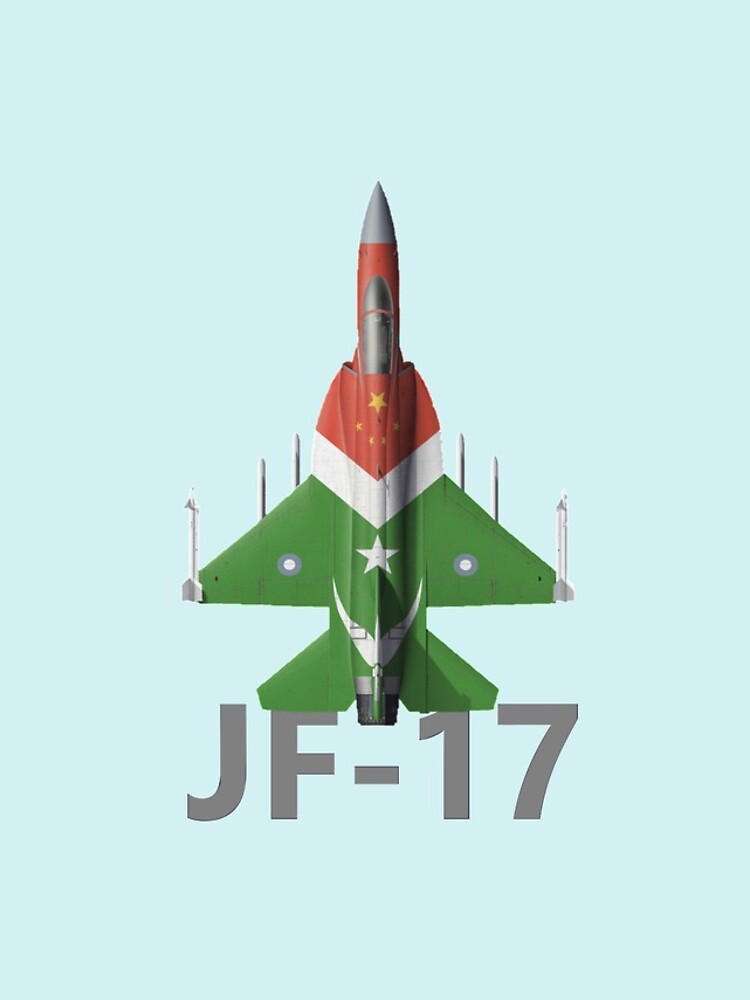This image features a detailed graphic illustration of a fighter jet identified as a JF-17. The jet displays a striking color palette: primarily green with red accents at the top, yellow stars reminiscent of a Chinese flag, and a distinct white "V" shape in the middle. Additional features include a white stripe and various elements protruding upwards, suggestive of missiles. The aircraft, oriented upwards and appearing missile-like, stands against a light blue background. Grey text at the bottom of the vertically oriented poster reads "JF-17." The composition and intricate design suggest this is a stylized, artistic rendering rather than a real-life photograph.